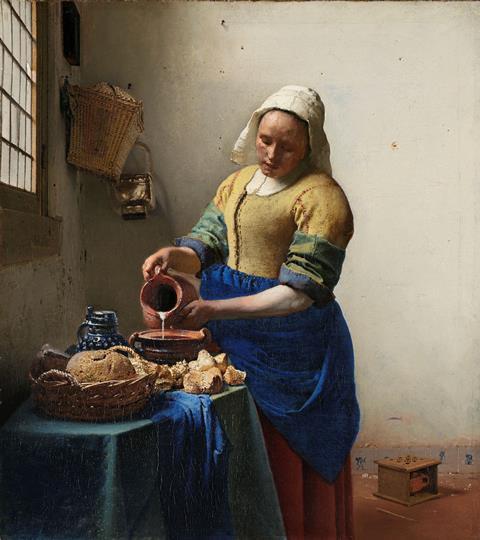The painting depicts a Dutch woman, reminiscent of Vermeer’s style, engrossed in her task of pouring a white liquid, perhaps milk or cream, from an earthenware pitcher into a bowl. She wears a traditional white headdress that frames her face and extends behind her head. She is adorned in a yellow bodice with a distinctive black stripe down the middle and green-gray details around her biceps, paired with a royal blue dress. Her stout figure suggests she is slightly overweight.

The scene is set in a room with light cream-colored walls, on which hangs a basket on the upper left quadrant. The far-left side of the painting features a wooden-framed window with multiple panes, allowing light to filter through. The woman stands by a small table covered with a green tablecloth and a blue towel draped over it. On the table rests a basket containing bread and several bread chunks scattered around.

In the background, on the floor to the bottom right, there is a light brown wooden box. The overall ambiance and details, including the woman's attire and setting, allude to a serene, everyday moment in a rustic, possibly 18th-century Dutch household. The woman’s expression is calm and focused, adding to the painting's sense of quiet diligence.